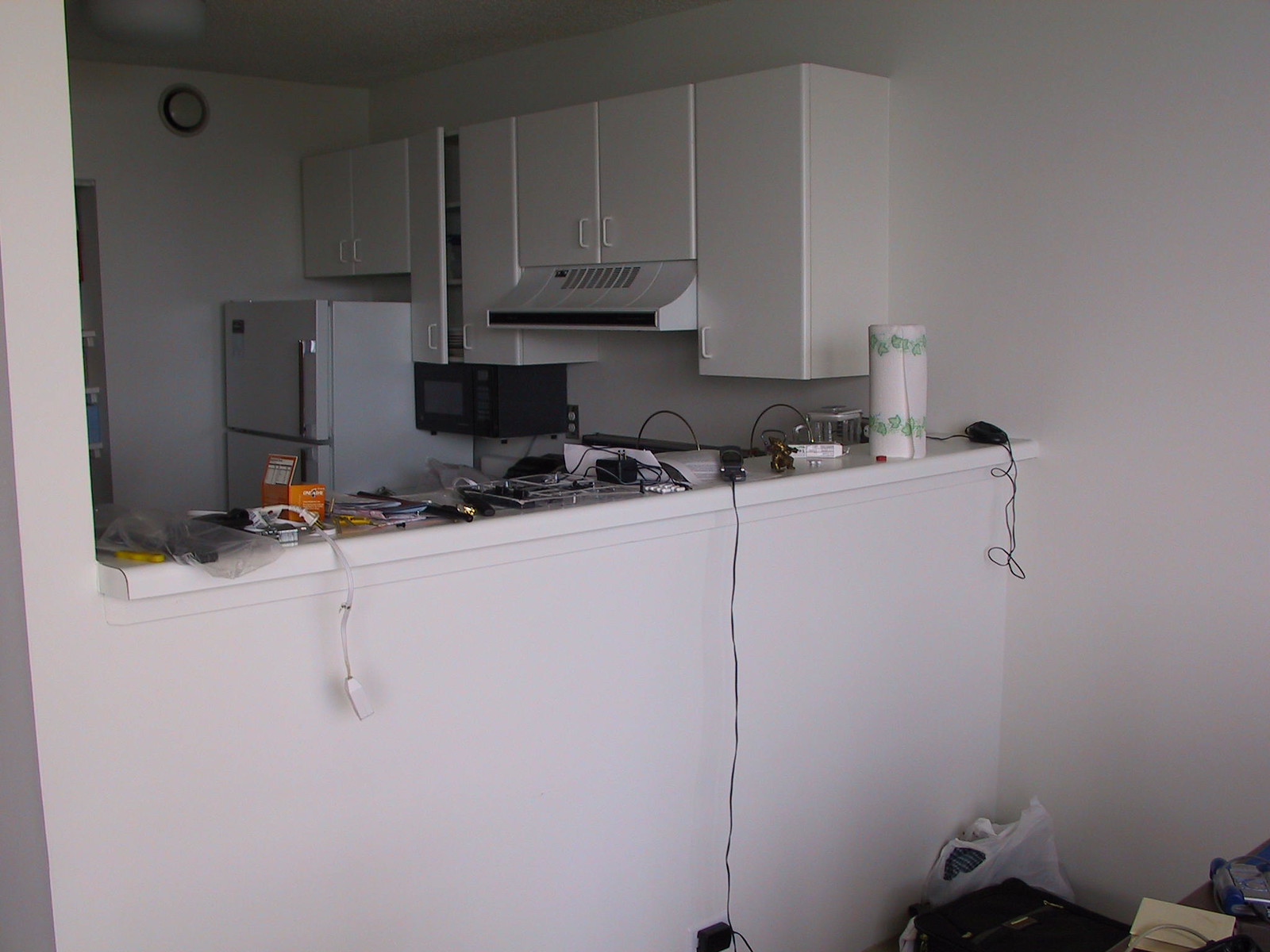In the image, Timmy stands in the kitchen, prominently featuring a white wall to the left. At the top-left corner, a kitchen clock is mounted. Overhanging cabinets are seen with various knick-knacks and gadgets placed around, and some items even hang from the ceiling. Near the center right, a phone is charging amidst other small electronic devices in the background. The back wall is also white, with a roll of paper towels positioned towards the middle right. A black microwave sits on the back left counter. At the bottom right, grocery bags filled with items are visible. The entire scene presents an eclectic mix of household items and devices, capturing a typical day in the kitchen.